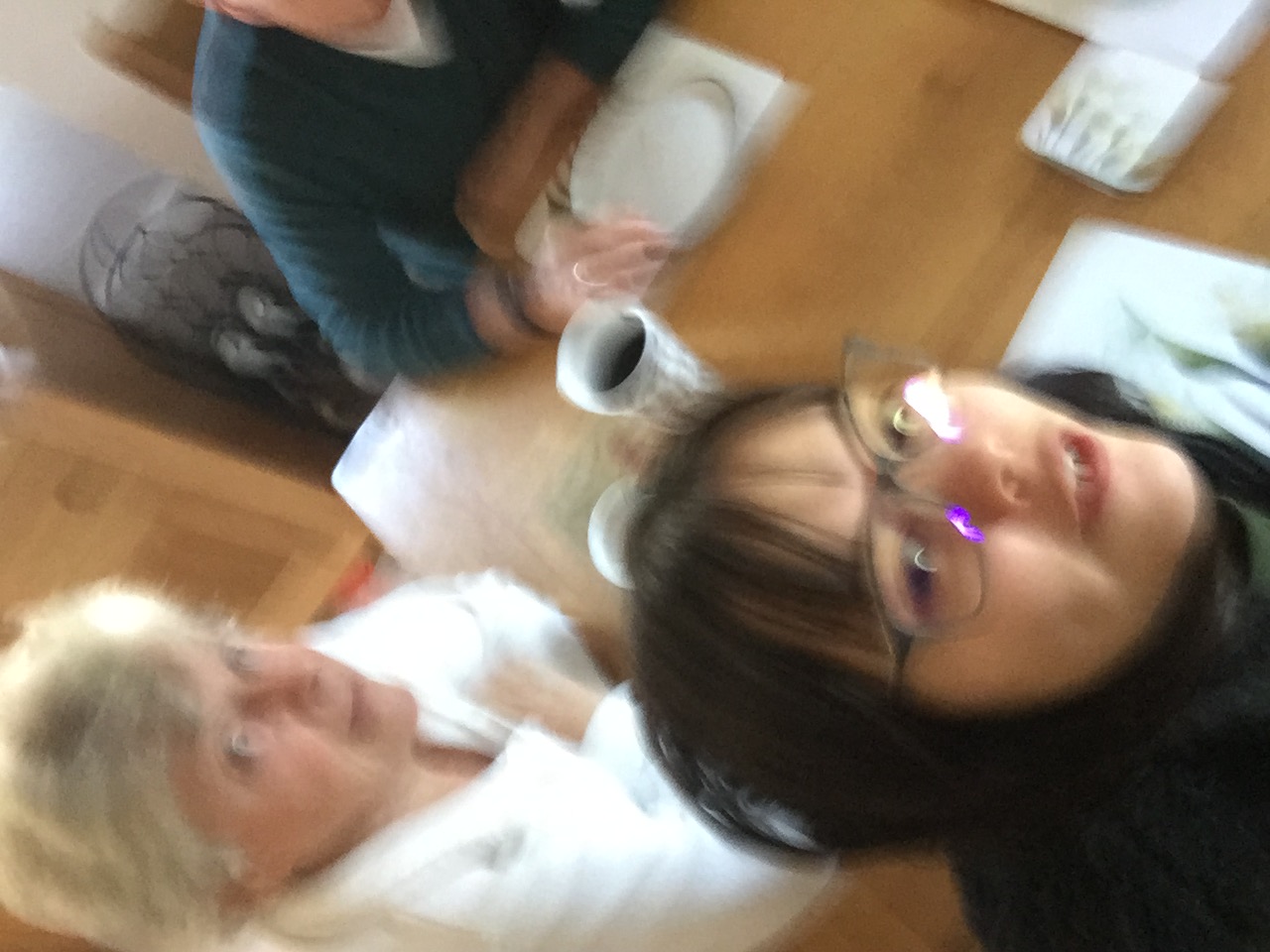A blurry image captures three individuals seated at a light-colored wooden table, likely engaged in a meeting or casual gathering. In the foreground, a young woman with dark brown hair, bangs, and glasses, dressed in a dark shirt, is visible in the bottom left corner. She has a white paper in front of her on the table. Positioned slightly behind her and to the top left is an older woman with short white or gray hair, wearing a white jacket or shirt, sitting with both elbows on the table. Across from the young woman, in the upper right-hand corner, the left-side shoulder of a man in a dark sweater wearing a watch is partially seen. The man has a plate in front of him while the older woman has two small white cups. In the background, wooden cabinetry matching the table is noticeable, along with a white shelving unit. The setting appears to be warmly lit, with several elements like a white bowl and possibly a bird cage adding to the casual ambiance.